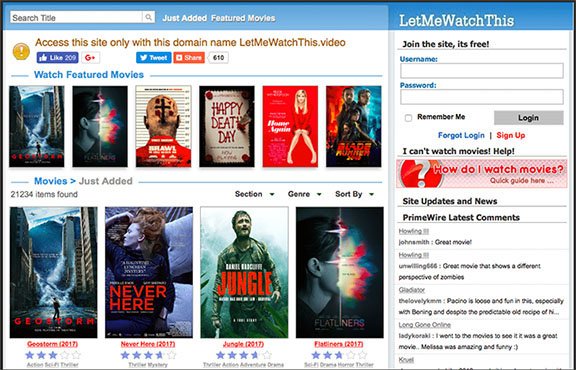The screenshot is of a website named "Let Me Watch This," displayed in a landscape orientation within a web browser. At the top of the webpage, a blue menu bar spans across the screen, featuring a white search bar with black text that reads "Search title." Adjacent to the search bar, white text options include "Just Added" and "Featured Movies."

On the right-hand side of the webpage, there is a vertical column dedicated to user login information. This section starts with the website's name, "Let Me Watch This," in white text. Below it, a prompt reads, "Join the site, it's free," followed by text boxes to input a username and password, a checkbox for the "Remember Me" option, and a grey login button. Additional links for "Forgot Login" and "Sign Up" are also visible, along with some brief messages from their PrimeWire messaging board.

The main content area on the left side of the screenshot displays various movie results divided into two sections. The top section, labeled "Watch Featured Movies," showcases covers for six different films. The bottom section, titled "Movies Just Added," indicates that a search has yielded 21,234 items. This section presents the posters for four movies, complete with star ratings, their titles, and the years they were released.